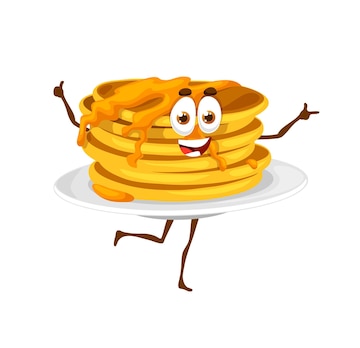This charming cartoon features a stack of six golden-brown pancakes, neatly arranged on a simple white plate. Each pancake is drizzled with rich, flowing maple syrup that cascades deliciously down the sides. Adding to the whimsy, the stack of pancakes is anthropomorphized with big, expressive eyes and a wide, cheerful mouth. From beneath the plate, two black, sticky legs protrude, one of which is playfully kicked back. The stack is equipped with two animated hands: the left hand offers an enthusiastic thumbs-up, while the right hand points off to the right. Set against a plain white background, this lively illustration exudes a sense of joy and positivity, capturing the essence of a happy, animated stack of pancakes on the move.